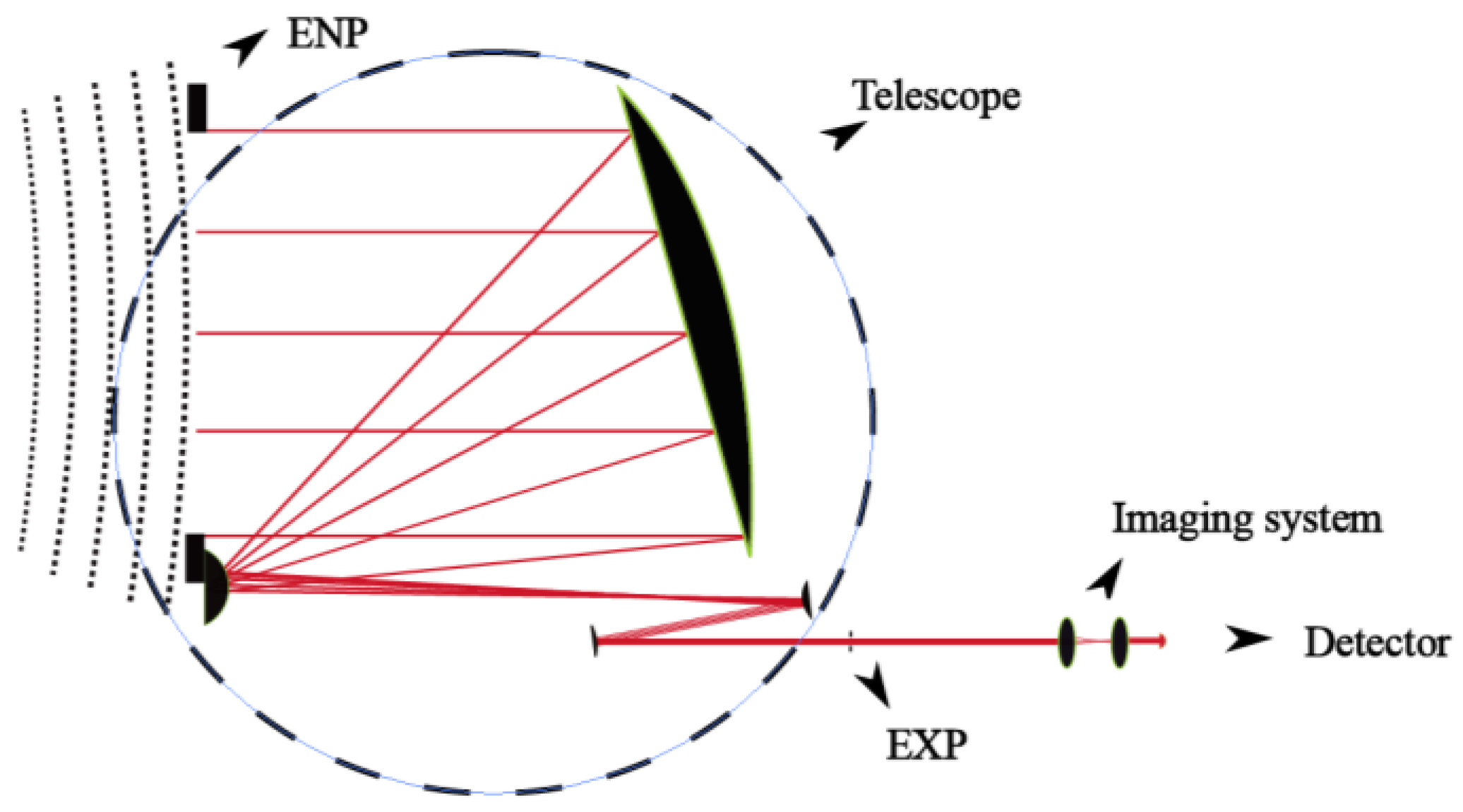This is a detailed diagram of an imaging system, set against a white backdrop. Central to the image is a large circle made up of alternating baby blue and black dotted lines. Inside this circle, a complex network of red lines forms Z-shaped patterns, crisscrossing both vertically and horizontally. These red lines appear to emanate from the top and progress downwards, pointing toward a central circular figure, identified by a nearby arrow as a telescope. 

On the periphery of the circle, there are labels in black capital letters: "ENP" at the top left, "telescope" at the top right, and "EXP" at the bottom right. At the bottom of the circle, a red line extends outward toward a label that reads "detector." Additionally, there is an arrow pointing upward, and the words "imaging system" are featured prominently above. The entire diagram is meticulously detailed, emphasizing the structure and function of the imaging system.